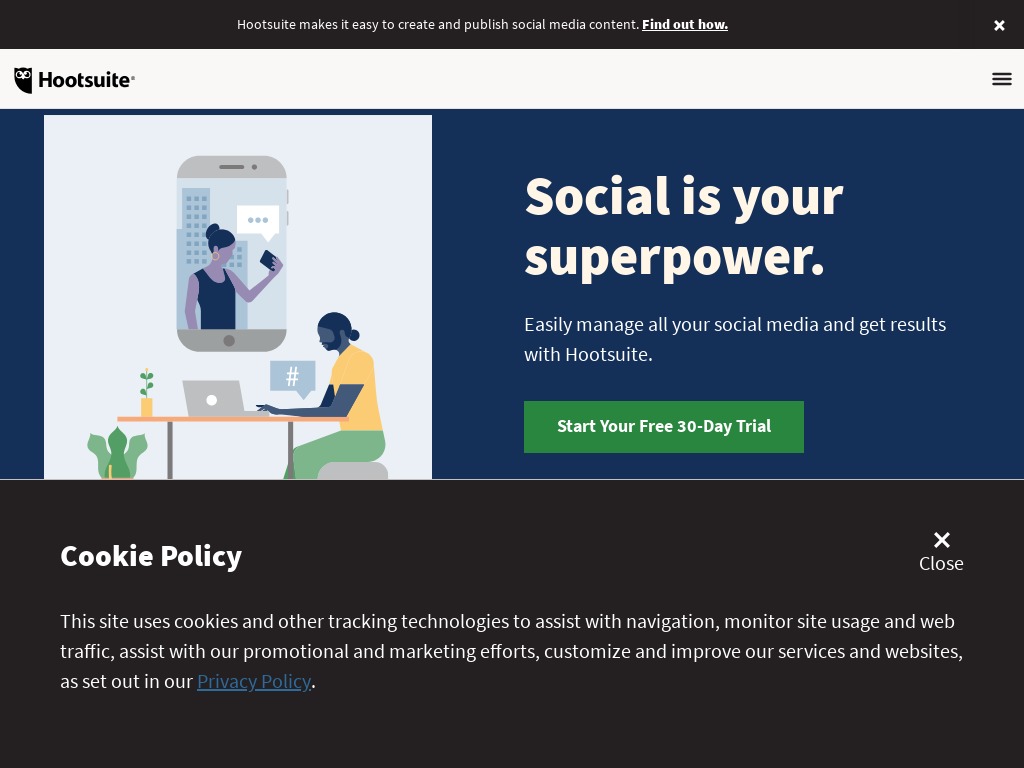The image depicts a screenshot of the HootSuite website. 

At the top of the image, there is a black bar with white text that reads, "HootSuite makes it easy to create and publish social media content." Next to this text is an underlined hyperlink stating, "Find out how."

Below the black bar, there is a horizontally aligned white bar approximately an inch thick. On the far left corner of this bar is the HootSuite logo, featuring the name "HootSuite" and its owl symbol. On the right side of this bar is the menu button.

The main section of the image features a large, navy blue rectangle background. On the left side of this background is a white box containing images. Inside the white box, there is a picture of a woman displayed within the frame of a white smartphone. The woman is standing in an urban environment with buildings in the background, looking at her own phone, which has a chat bubble above it. Below this image, there is a picture of a person sitting at a desk wearing a yellow shirt and green pants, working on a laptop.

On the right side of the blue section, the text reads, "Social is your superpower. Start your free 30-day trial."

At the very bottom of the image, there is a cookie policy pop-up notification.